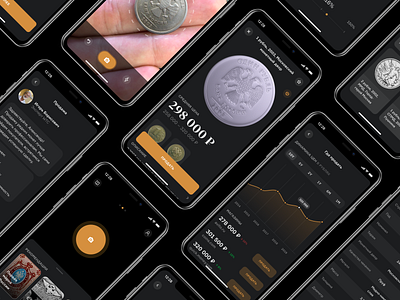This image, taken from a top-down perspective, shows a horizontal arrangement of smartphones against a black background, organized in neat rows leaning to the right. There are parts of eight to ten smartphones visible, each with slender grey edges, contributing to a sleek, modern aesthetic. The majority of the phone screens have black backgrounds adorned with various financial graphics, such as stock graphs in vibrant orange and images of coins in gold or silver hues. One phone prominently displays a silver coin with the inscription "29800P," while another features an image of a hand holding a coin with three fingers, palm up. Interspersed among the phones, there are fragments of white text that are too small to decipher clearly, except for the aforementioned "29800P." Some phones also have yellow buttons and additional numerical data, which likely pertains to financial or stock market information, possibly even cryptocurrency like Bitcoin. Overall, the image conveys a sense of financial analysis or trading, highlighted by the graphs and coin imagery.